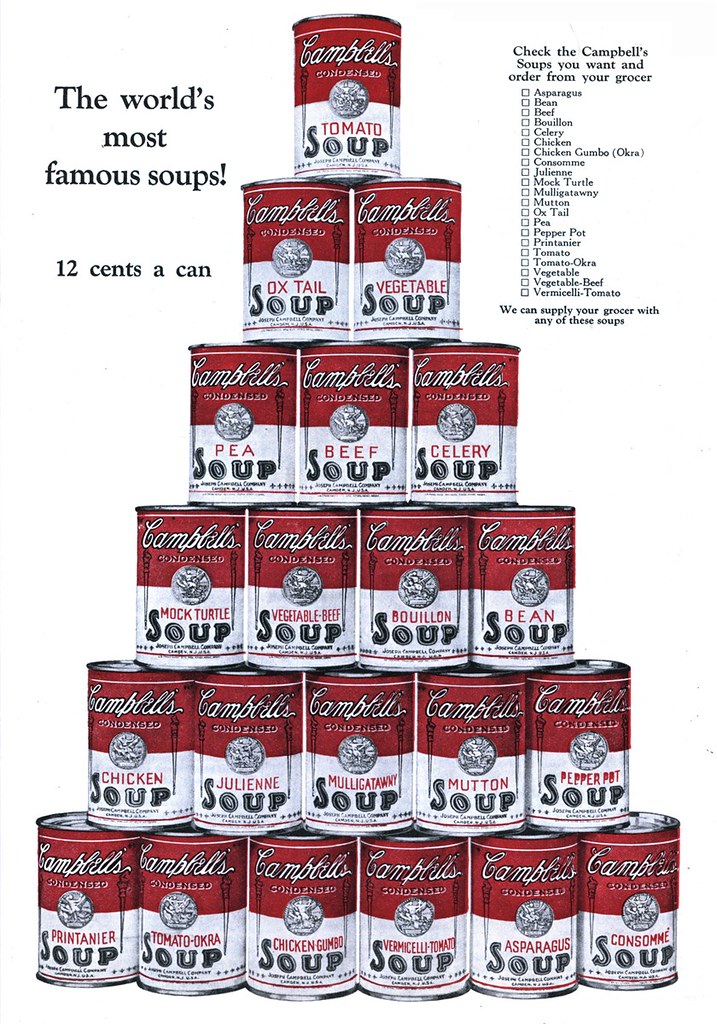This vintage advertisement for Campbell's Soup features an intricately stacked pyramid of soup cans, showcasing a diverse array of flavors. The pyramid starts with six cans on the bottom row, then progresses upward with five, four, three, two, and finally one can at the top. Each can is distinct, with red tops and white bottoms, adorned with white "Campbell's" lettering, black "soup" text, and red descriptors identifying the flavor. The pyramid includes varieties such as tomato, beef, celery, pea, bouillon, bean, and mock turtle, among many others. Flavors listed range from common ones like tomato and chicken to unique choices like multigottany and pepper pot. The background is white, with text on the left proclaiming "the world's most famous soups" and "12 cents a can," indicating the advertisement's age. To the right, a detailed list invites consumers to check the Campbell’s soups they want to order from their grocer, covering an extensive alphabetical lineup that can satisfy any palate. This comprehensive ad emphasizes Campbell’s ability to supply any of these flavorful soups to grocers, asserting its market prominence and variety.